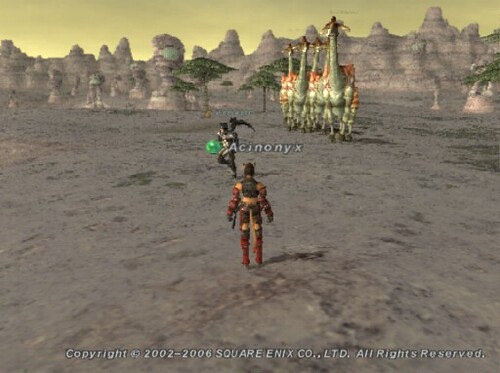In this image from a video game by Square Enix Corporation, set between 2002 and 2006, two adversaries face off on a barren desert plateau. The first character is clad in a striking burgundy outfit with yellow accents and black details, clearly prepared for battle. Opposing him is a figure dressed in an imposing black and gold ensemble. Behind the black-and-gold character, four colossal creatures, resembling a hybrid of giraffes and camels augmented in size, stand menacingly. These creatures appear to have red saddles, adding a vivid splash of color to their formidable presence. The background showcases an intriguing geological formation of stratified rock, reminiscent of the Buttes found in the Western United States, further enhancing the arid, rugged ambiance of the scene.